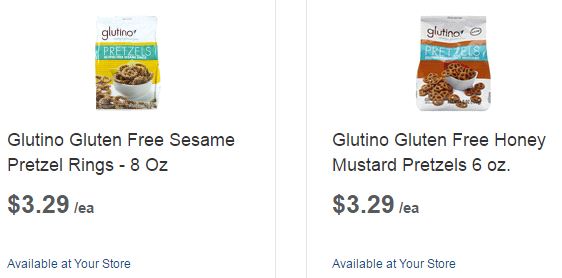The image consists of two side-by-side packages of gluten-free pretzels from the brand "Glutino." 

On the left, the package features a white top section displaying the brand name "Glutino" in bold letters. Below it, a yellow background is adorned with a blue stripe that reads "pretzels." The front of the package showcases a white ceramic dish filled with sesame pretzel rings. The label indicates: "Glutino Gluten-Free Sesame Pretzel Rings, 8 oz," priced at $3.29 each and available at your local store. 

On the right, the package also has a white top section with the "Glutino" brand name prominently displayed, along with a blue stripe that says "pretzels." The rest of the package has an orange background depicting honey mustard pretzels spilling out of a white ceramic bowl. The label reads: "Glutino Gluten-Free Honey Mustard Pretzels, 6 oz," also priced at $3.29 each and available at your local store.